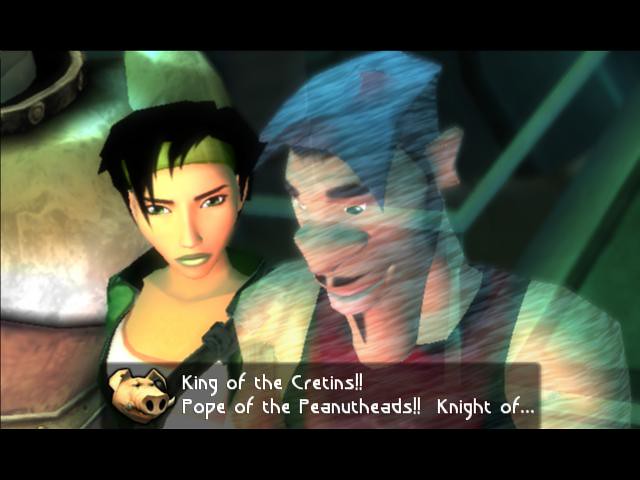The image is a screenshot from a video game, featuring two characters in the foreground with black borders at the top and bottom. On the left side of the frame is a focused female character with short, black hair, styled with a lime green bandana and bangs. She has olive, almond-shaped eyes, a long nose, a diamond-shaped face, and green lips. She's dressed in a white tank top covered by a green sweater or jacket. To her right is a semi-transparent, slightly blurred male character with bluish hair fashioned into an undercut with a flat top and a side bang. He sports a goatee, a pointy mustache, and is wearing a red vest over a white t-shirt. This man appears almost ghostly or holographic. Below them, there is a transparent dialogue banner featuring a pig icon on the left and text that reads: "King of the Cretins!! Pope of the Peanut Heads!! Knight of..." The rest of the background is indistinct and filled with vague shapes.